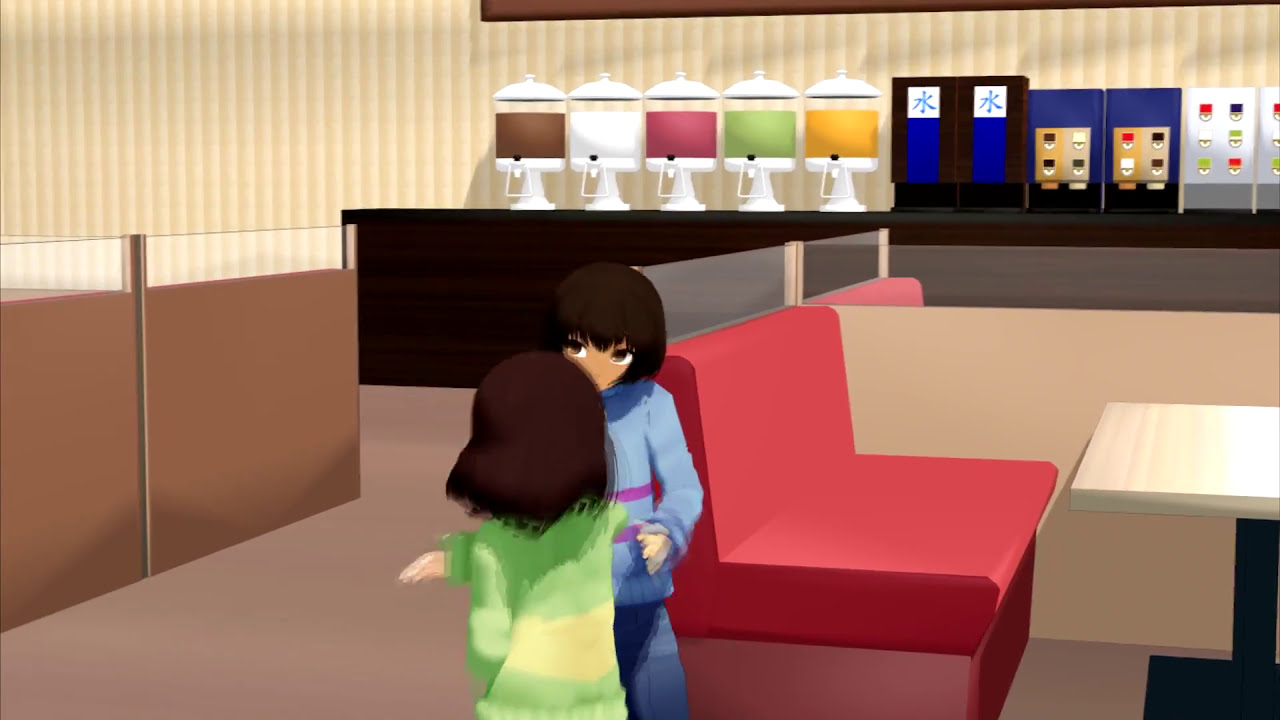This color cartoon illustration depicts a lively restaurant scene with two human figures at the center. The figure closest to the viewer is a girl with long, straight brown hair wearing a green dress with yellow stripes. She appears to be in motion, as if she has just swung her right arm, hitting the person in front of her. The startled figure facing her has chin-length straight brown hair, wide brown eyes, and is dressed in a long-sleeved blue shirt with purply-pink stripes along with blue pants. 

They stand near a restaurant booth to the right, characterized by its pink seats and a wooden table with glass dividers. More booths are visible behind them, each separated by wooden dividers with glass tops. To the left, additional dividers mirror this design. The background features a brown and beige vertically striped wall, complemented by a black counter adorned with various drink dispensers displaying a colorful array of beverages, including shades of brown, white, pink, green, and yellow. The scene is rich in detail, capturing the energetic ambiance of the restaurant.